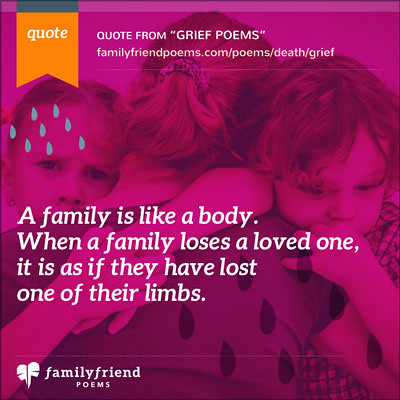The image is a poignant advertisement with a magenta-tinted background. It features a woman viewed from behind, her brown hair pulled into a ponytail, being embraced by two children. On her left is a little boy with his hand in his mouth, looking down in sorrow, while on her right a little girl stares directly at the viewer, her expression conveying deep devastation. Superimposed over these figures are blue and black teardrops, symbolizing grief. The top of the image displays an orange banner with the text, "Quote from Grief Poems, familyfriendpoems.com/poems/death/grief." Centrally, in white lettering, a profound quote reads, "A family is like a body. When a family loses a loved one, it is as if they have lost one of their limbs." The bottom left corner of the image features the logo of Family Friend Poems.